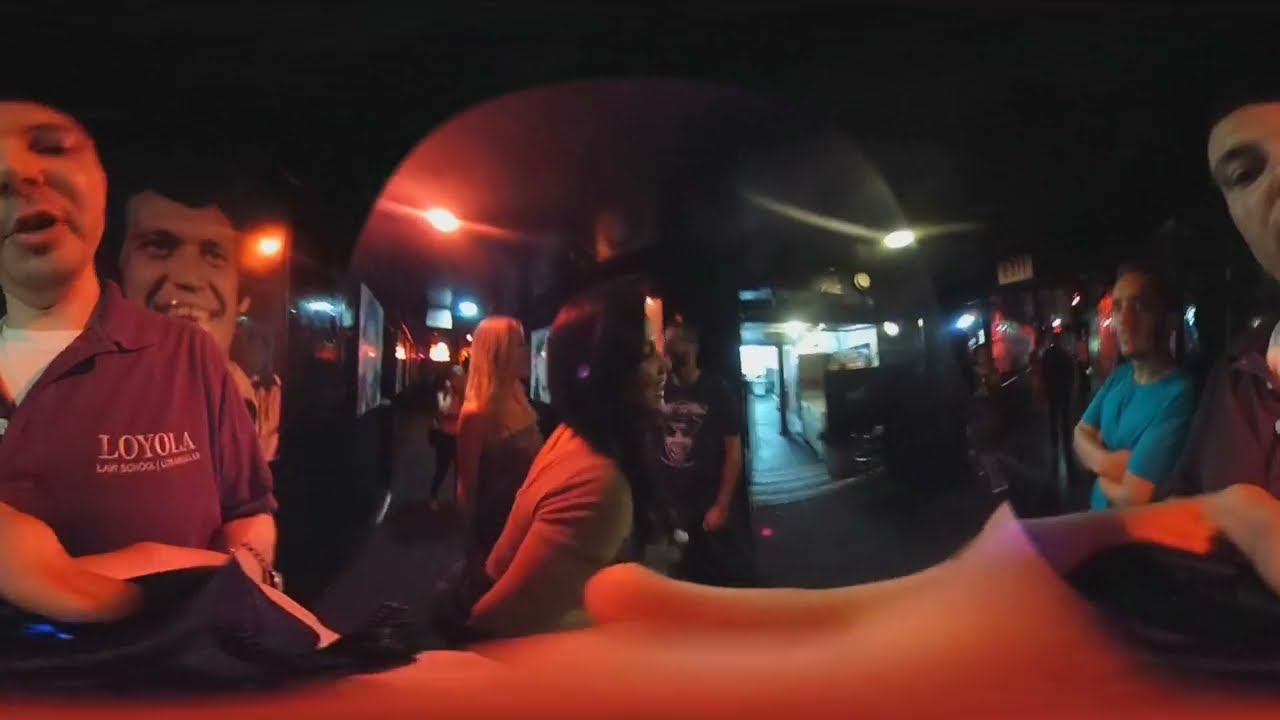The image depicts a lively group of people, likely at an indoor bar or dance club, characterized by a dark ambiance. Prominently, there is a woman to the right in a maroon shirt. To her left stands a man in a blue shirt with his arms crossed, and next to him, a woman with long black hair. Behind her, another woman with long blonde hair is visible. The background is dimly lit with some scattered lights, revealing blurred figures and adding to the bustling atmosphere. The ceiling is black, matching the dark floor and contributing to the overall dimness. In the furthest background, an entryway is faintly illuminated, suggesting an outdoor view. The lower and upper edges of the photo are bordered by black bars, framing the scene. Despite the lack of visible drinks, the setting and the crowd's demeanor imply a social and festive environment.